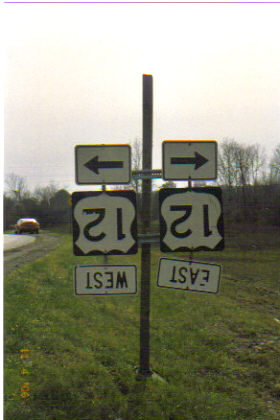In this outdoor photograph, set against a winter or early spring landscape with bare trees and a gray sky, the main focal point is a signpost standing prominently in the grass by the roadside. The signpost consists of a sturdy metal tube rising vertically, with two horizontal steel bars supporting directional street signs. These rectangular signs, intended to display route numbers and directional arrows for "East" and "West," are conspicuously upside down—most likely due to a loose top screw. This unusual orientation misleadingly alters an "East" arrow to point "West," and a "West" arrow to point "East," while the "12" route number appears as an odd "51." To the left of the signpost, part of the roadway is visible, along with a parked car. Adding a touch of color to this otherwise muted scene, a few yellow dandelions are scattered in the lower corner of the grassy area.